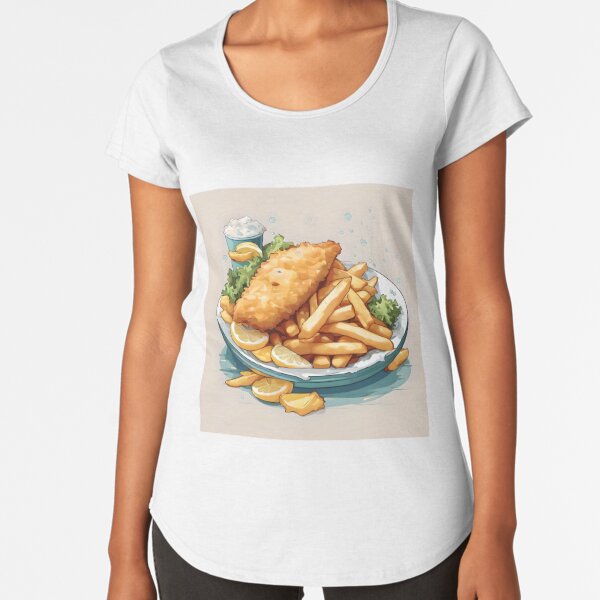The image depicts a Caucasian woman dressed in a white short-sleeve scoop neck t-shirt and black pants, possibly yoga pants. In the center of her t-shirt, there is a tan square featuring a detailed illustration. The illustration appears AI-generated and shows a blue plate with a piece of fried fish, several French fries, and lemon wedges artfully arranged around it, with some pieces falling off the plate. Additionally, there's a bit of lettuce underneath the fish and fries. To the left in the background, a blue cup filled with a white foamy liquid can be seen. The image only includes the woman from her neck down to her arms, without showing her head or fingernails.